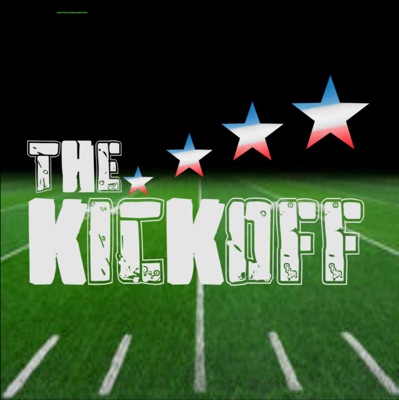This square-shaped digital poster features a striking two-part background: the upper half is completely black, while the lower half showcases a vividly green football field marked with yellow and white lines. Dominating the center of the image, in bold white block letters, are the words "THE KICKOFF." These words span two lines, with "THE" on the top line and "KICKOFF" below it, both left-justified. Emerging from the top of the letter 'C' in "KICKOFF," a series of four stars extends upward and to the right, increasing in size along the way. These stars are tri-colored: red at the bottom, white in the middle, and blue at the top, contributing to a visually striking and patriotic theme.